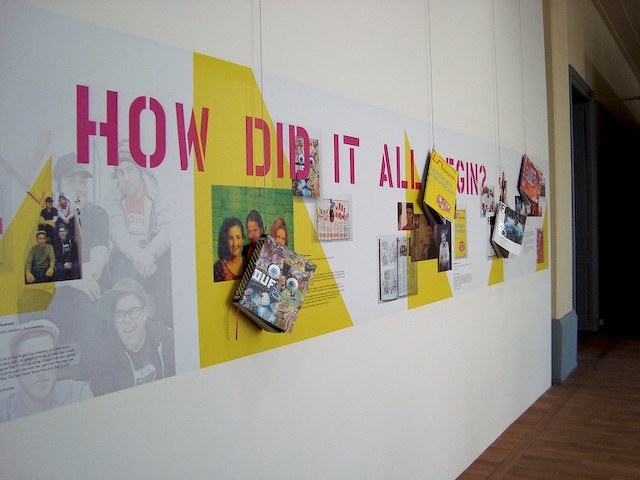This photograph captures a white wall in a historical setting, possibly a museum or school, adorned with a wall mural. At the top, bold pink letters spell out "How did it all begin?" Beneath this question, various items and images are arranged in sections along the wall. Starting from the left, there is a projected photo featuring a group of boys, though the image is partially cut off. To the right of this, more artwork is displayed, including a picture with girls and a series of books, the first of which prominently features the name "Duff" and has a yellow background. As you move further right, additional images of people become less distinct, interspersed with books in different colors, such as yellow and orange. The display continues to the right, where it meets a hallway with an open door, suggesting that the mural might be part of a larger exhibit.